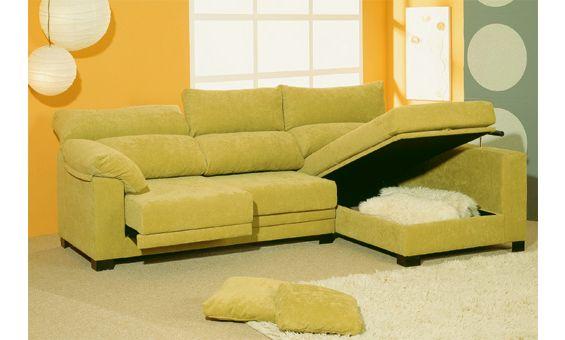This image, a realistic photograph with an almost surreal quality, depicts a potentially showroom or living room scene. The room features a vibrant color scheme: the back left wall is an orange-gold hue, while the right wall is a distinctive green adorned with large pale green circles. Centrally located on the back wall is a white window divided by light beige grid lines into nine panes, letting in natural light.

In the middle of the room is a multifunctional, L-shaped couch in a yellowish-tan color. The couch includes a chaise end on the right side that lifts to reveal storage space, which currently holds white shag blankets or towels. Another section of the couch can recline, adding to its versatile design. There are two beige throw pillows, matching the couch, positioned on the fluffy white carpet on the floor, which itself rests atop a light beige main carpet that covers the entire room.

Two round, white paper lanterns hang as light fixtures from the ceiling on thin wires, adding a whimsical touch to the decor. Various elements like the suggested storage functionality of the couch and the mixture of textures and colors create an inviting yet slightly peculiar atmosphere, enhancing the room's distinctive character.